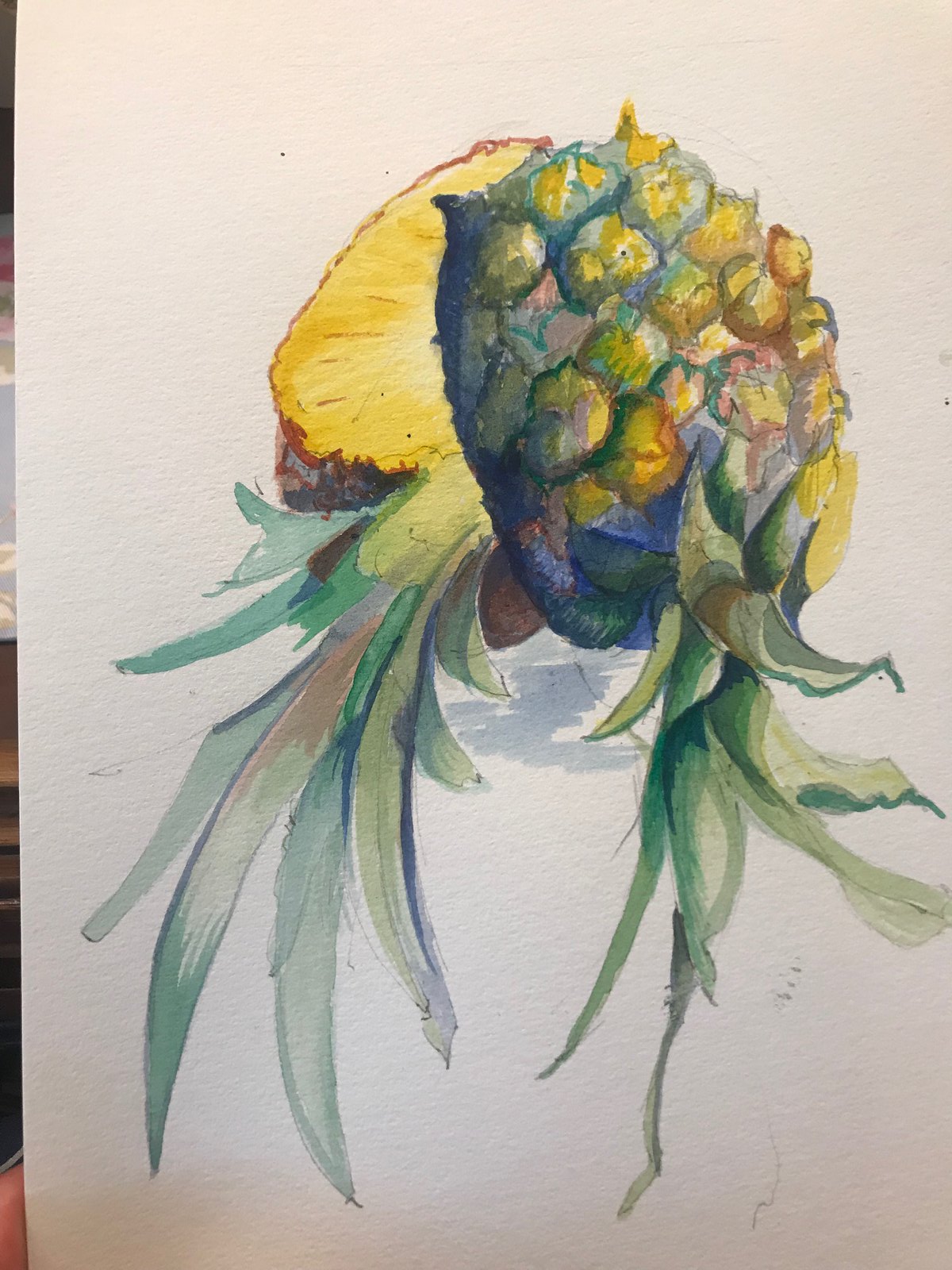This image showcases a watercolor-style painting on a white surface, depicting an abstract interpretation of pineapples cut in half. The left half of the pineapple features a yellow center, surrounded by a brown body, and is adorned with shades of dark and light green leaves, sprinkled with hints of brown. The right half displays the spiky top of the pineapple, rendered in varying tones of yellow, brown, and both light and dark green, along with green leaves tinged with brown as well. At the top of the painting, subtle white reflections contrast with faint, dirt-like scuff marks that are visible on the white backdrop. Delicate gray shadowing adds depth to the pineapple, enhancing its textured appearance.